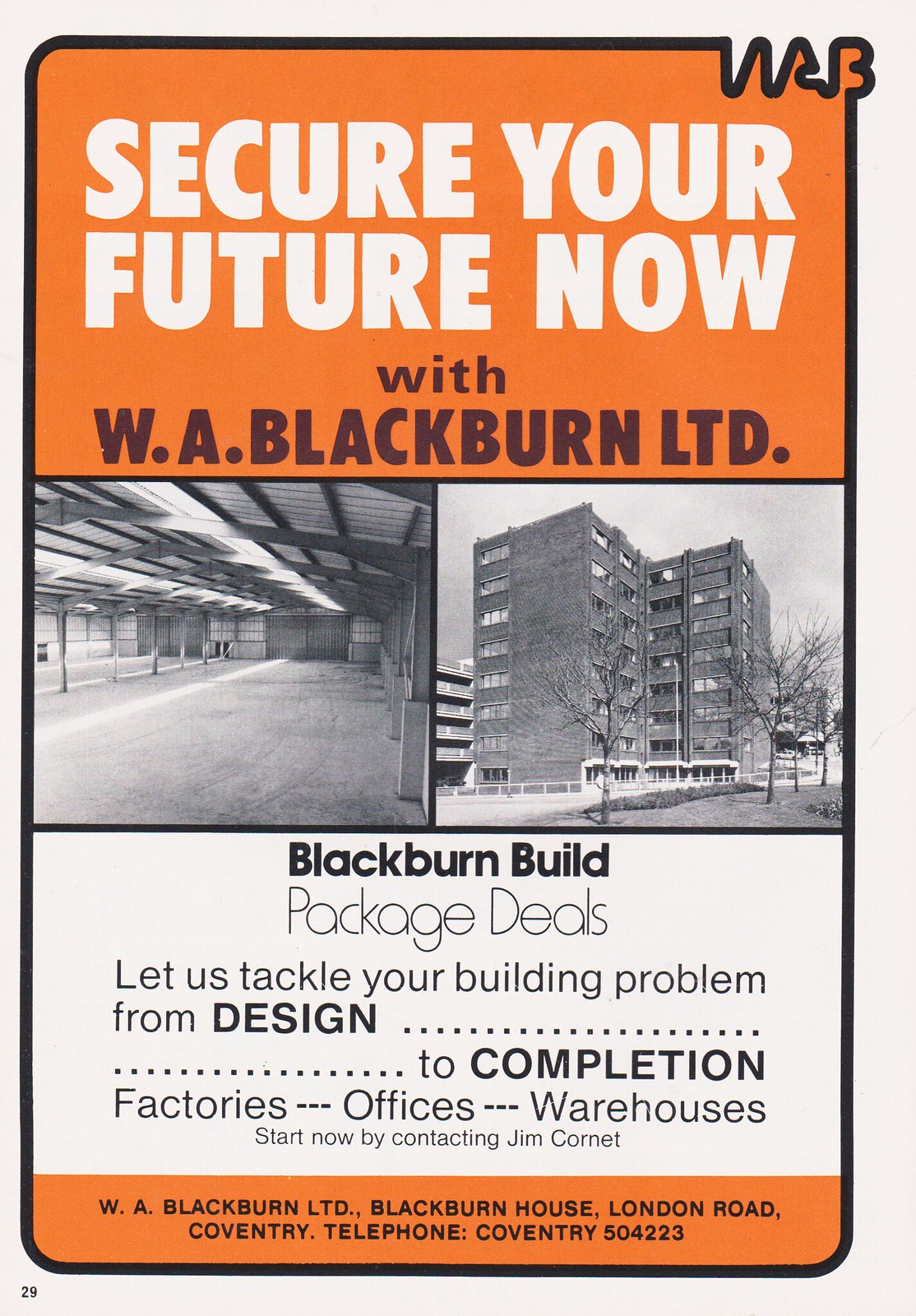This advertisement, likely from the 60s or 70s, features a prominent orange banner on a white or off-white background. The banner's white letters read: "Secure your future now with W.A. Blackburn Ltd." The ad includes black and white photographs showing both the interior of a warehouse and the exterior of a seven-story building. Beneath the images, the text states: "Blackburn builds package deals. Let us tackle your building problem from design to completion." It highlights their expertise in factories, offices, and warehouses. The bottom section of the flyer, also in an orange banner, provides contact details: "Start now by contacting Jim Cornett at W.A. Blackburn Ltd, Blackburn House, London Road, Coventry. Telephone: Coventry 504-223."